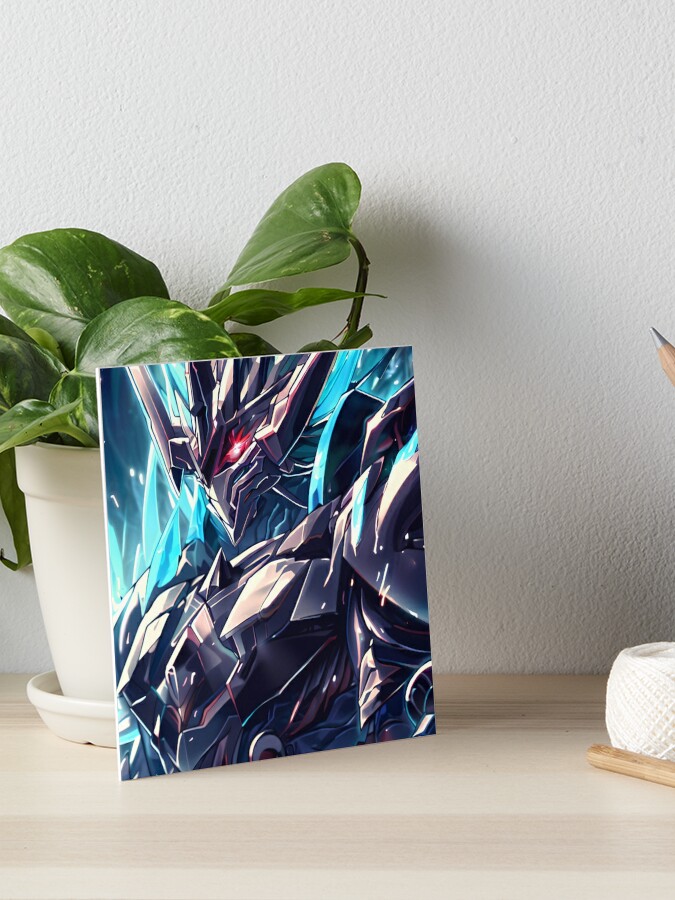The image features a painting primarily in a vertical rectangular format, positioned against a light gray wall. The painting, set within a smaller white rectangular canvas, leans against a white plastic plant pot that contains green foliage. It rests on a light grain wooden cabinet top. The artwork depicts a futuristic gray steel robot, visible from the chest up, with a distinctive V-shaped face and red glowing eyes. The robot's head design is reminiscent of a crown, and it boasts a massive metal chest with intricate armor detailing. Various shades of blue, resembling crystal spikes, compose the background. Additional elements in the image include a spool of white thread, a brown handle, and a silver pencil on the right side of the composition. The photograph seems to be taken directly in front of the setup, emphasizing the painting while capturing the indoor setting. The color palette of the scene includes light blue, dark blue, red, gray, silver, off-white, tan, beige, and dark green.